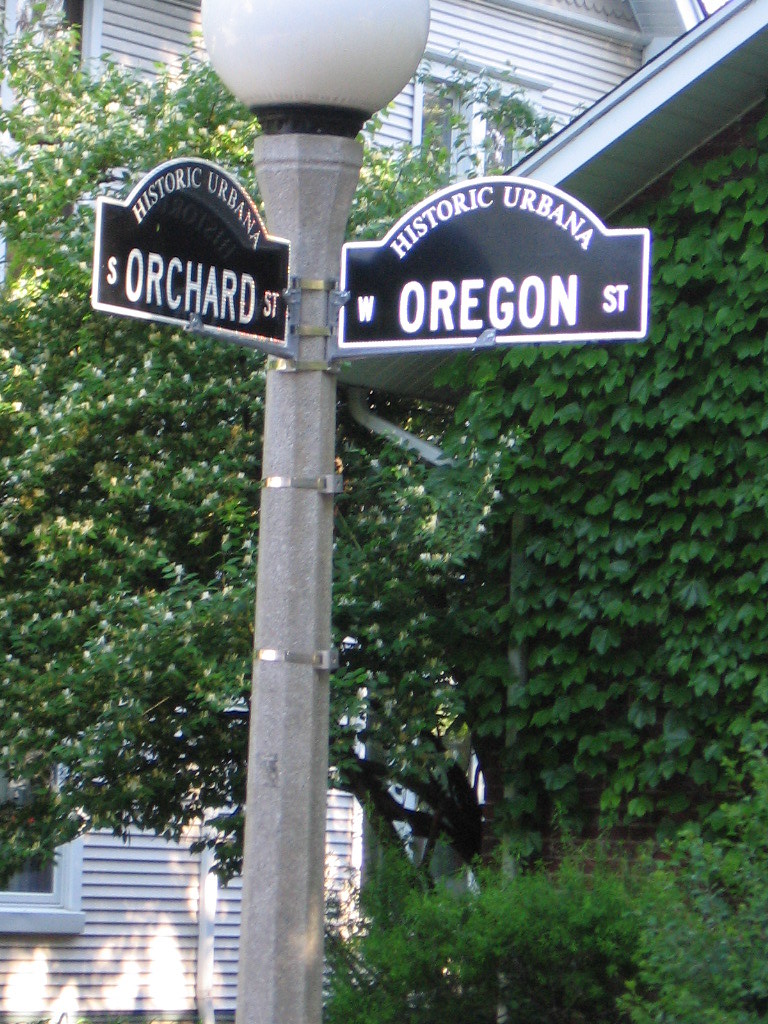The color photograph, taken outdoors in portrait orientation, captures a detailed view of intersecting street signs in a North American setting, specifically Historic Urbana. Dominating the scene is a unique, hexagonal granite lamp post that hosts the street signs. The sign facing the camera identifies "West Oregon Street," with the word "Oregon" prominently displayed in capital letters and flanked by smaller "W" and "S-T" texts. Perpendicular to this, a sign for "South Orchard Street" is affixed with metallic silver retaining straps. The street signs themselves feature a black background with reflective silver outlines that gleam in the daylight. Topping the post is a white, spherical light fixture.

In the background, a large, ivy-clad frame house stands adjacent to another, more traditional home, enriched by green foliage and tree cover, suggesting a spring or summer season. Gentle, ambient light filters into the scene, possibly indicating morning time, contributing to the tranquil, historical ambiance of the location.